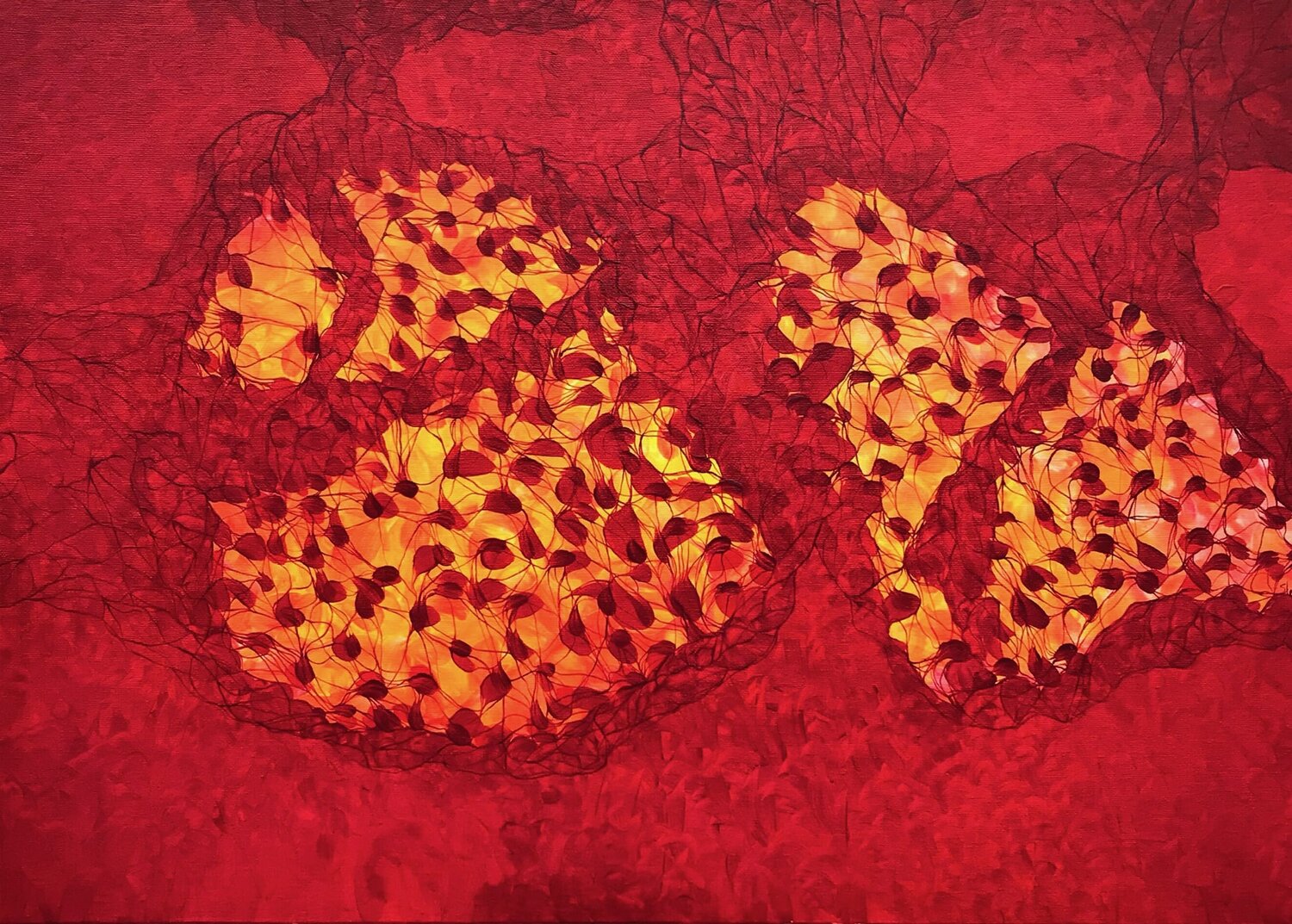The image is an abstract artwork dominated by various shades of red, ranging from light to dark. The background is a dynamic collage of intersecting curved lines, giving the appearance of a densely layered composition. Central to the piece are four distinct petal-like shapes in vibrant orange and yellow hues that sharply contrast with the surrounding red. These petals contain inner sections of red, echoing the background's color palette. The overall effect is reminiscent of fire or a floral motif, with orange highlights prominently shimmering through the predominantly red setting. The image appears to be a digital painting, rich in texture and complexity, devoid of any textual elements. The purposeful arrangement and interplay of colors reinforce its abstract nature, leaving its exact representation open to interpretation.